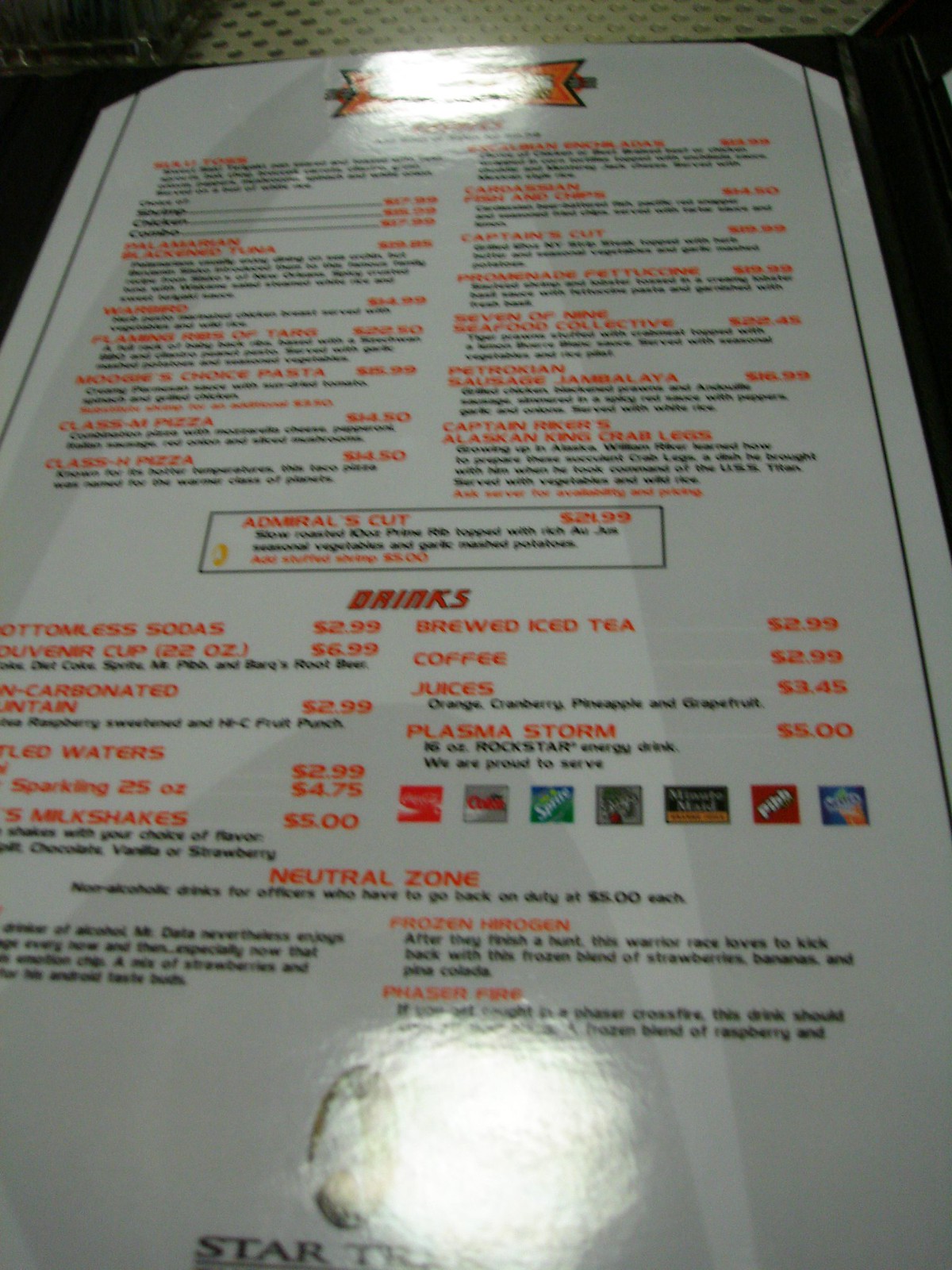This photograph captures a restaurant menu primarily colored in white, with most of the text in orange and black. The menu is laid out flat on a table, bathed in gentle sunlight streaming in from the top. Unfortunately, the restaurant's name at the top of the menu is unclear. 

In the middle section, there's a distinct box advertising a special, though the details are unreadable. Below this advertisement, there's a prominent section titled "Drinks." Listed towards the bottom of this section are various beverage options including brewed iced tea, coffee, and a selection of juices: orange, cranberry, pineapple, and presumably grapefruit.

An intriguing drink named "Plasma Storm" is mentioned next, accompanied by vibrant emblems. Further down, another item called "Neutral Zone" is listed, followed by a menu item described as "Frozen Something." 

At the very bottom of the menu, the words "Star Trek" stand out in black text, with a white element zipping past, adding a dynamic touch to the visual.